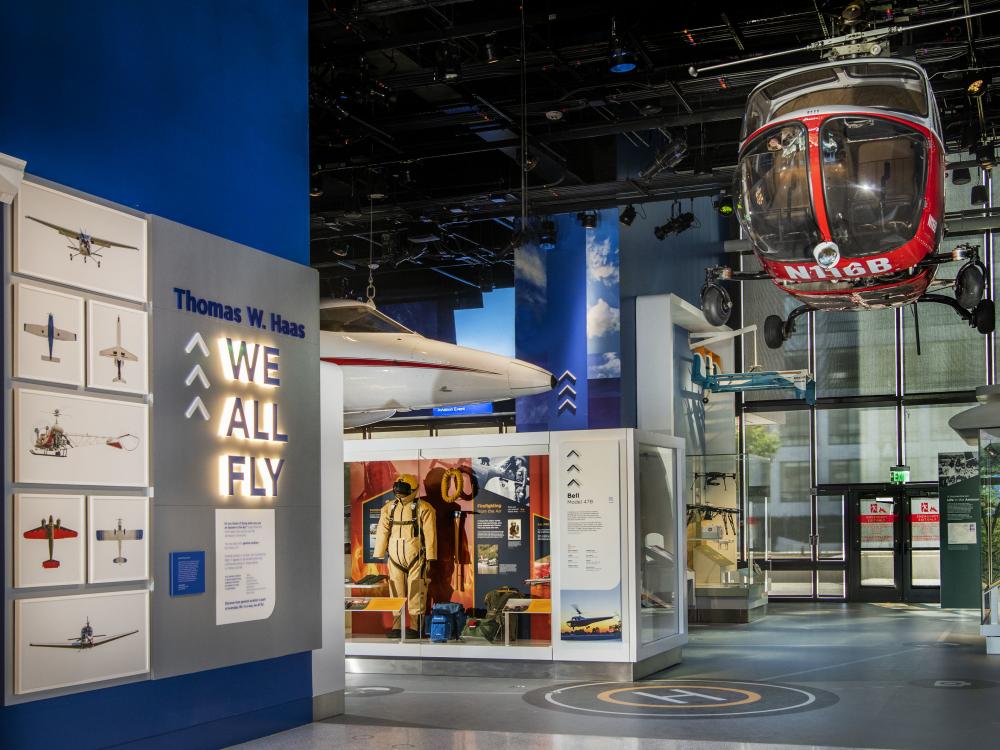The image depicts the interior of a flight museum, showcasing a variety of aviation exhibits. Dominating the scene is a red and white helicopter suspended in the upper right corner, prominently displaying the identification number N116B. It hangs above a marked helipad symbol, a large white ‘H’ in a circle on the concrete floor. The museum features a vibrant blue wall to the left, emblazoned with "Thomas W. Haas. We All Fly," and adorned with photographs of various single-wing aircraft and biplanes. Near this wall, there's a detailed display with a full flight suit, encased in a glass cabinet, and surrounding informational boards. Alongside this, additional exhibits display gear, backpacks, and further aviation information. The ceiling is intricate, with visible ducts, rigging, and directional can lights illuminating the displays below. A significant architectural feature in the background is a large glass wall with double doors leading outside, alongside which is an exit sign above a doorway with red writing. Further adding to the aerial ambience, the nose of a suspended jet is visible from above, completing the detailed and immersive exhibit environment.